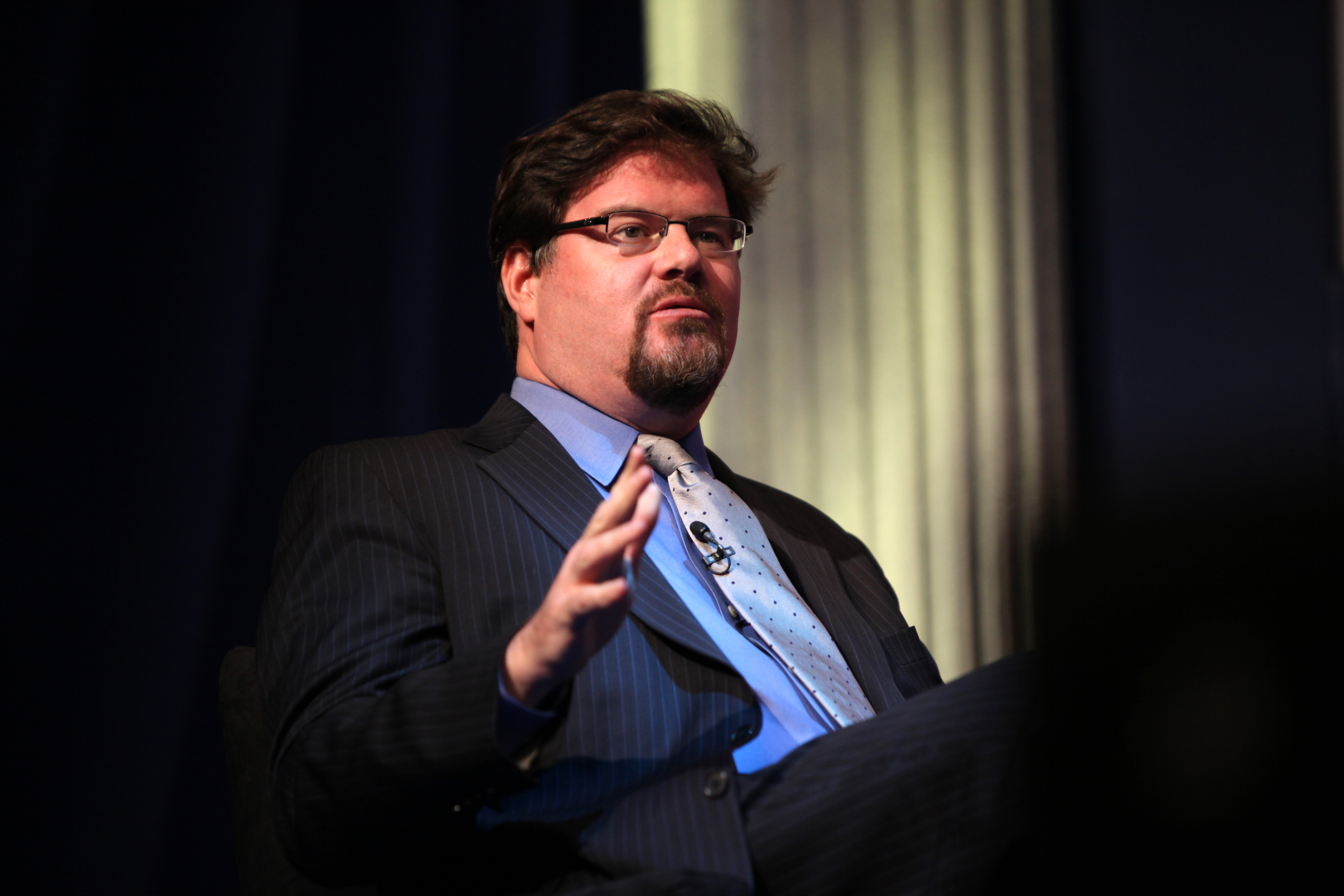A portrait photograph features a Caucasian gentleman sitting, possibly engaged in conversation. He is positioned in the lower part of the image, with his legs partially visible, seemingly crossed, and holding one hand out in front of himself, palm facing his thigh. The man is dressed in a dark suit, potentially black denim or pinstripe, with the jacket unbuttoned. Underneath, he wears a light blue collared shirt paired with a tie that appears silvery or white with black spots. 

The gentleman sports small, thin-framed glasses, which seem slightly undersized, balanced on the reddish-hued skin of his face. He has a goatee and medium-length brown hair. His teeth have a slight apricot tint. In the background, a slightly off-white or yellow backdrop, possibly featuring a white column, contrasts against navy blue curtains, suggesting an auditorium setting. The overall image is clear of any text or additional elements.